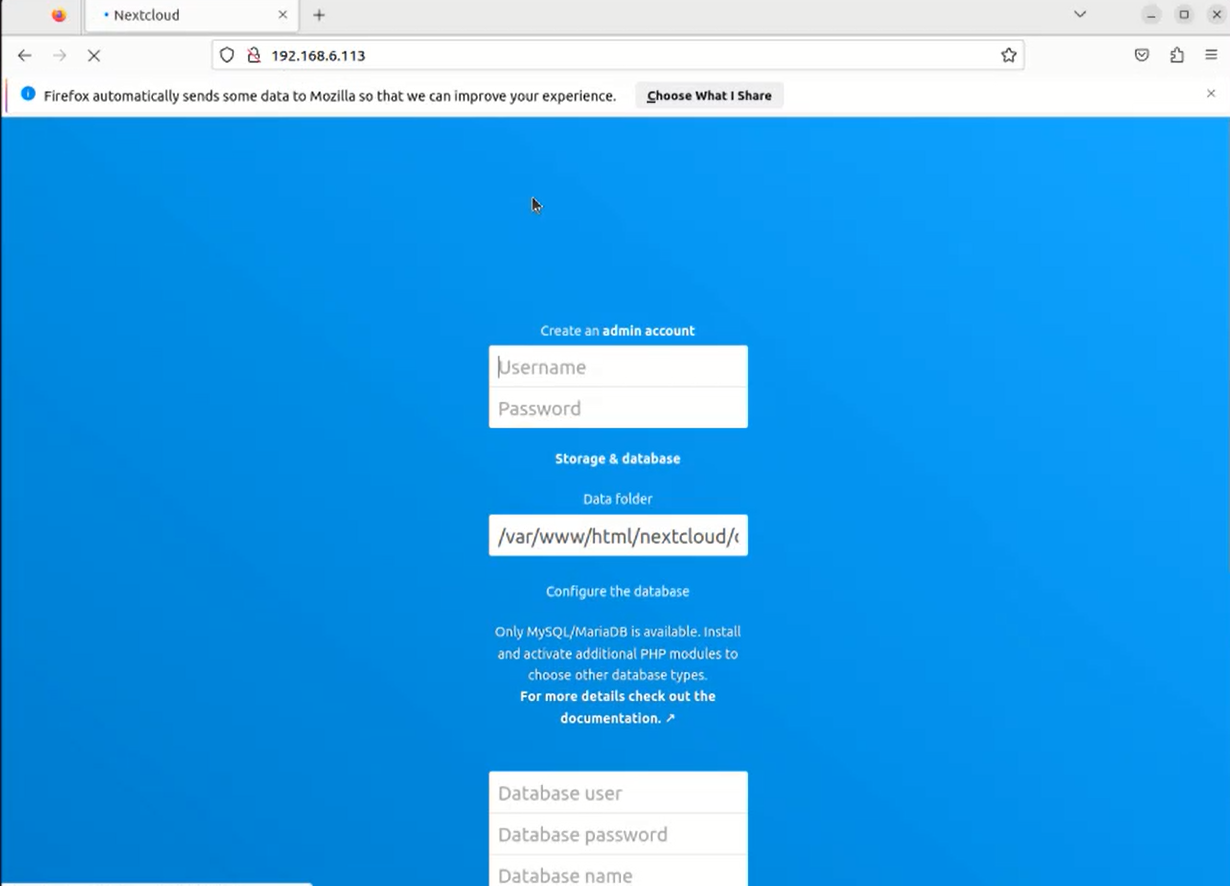The image features a computer screen displaying a Firefox browser window. In the top left corner, there is an open tab labeled "Next Cloud." Adjacent to it, towards the right, are the standard browser control icons: minimize, maximize, and close (X). Directly below this is the URL bar displaying a series of numbers, accompanied by a back arrow, forward arrow, and another X to its left. On the right side of the URL bar is a star icon followed by three additional computer-related icons. Beneath the URL bar is a message on a gray background stating, "Firefox automatically sends some data to Mozilla so that we can improve your experience. Here’s what I share."

Below this message, the screen transitions to a blue background, where the upper section prompts the user to "Create an Admin Account" with fields for entering a Username and Password. Underneath these fields, there's a section titled "Storage and Database," followed by another field labeled "Data Folder" that contains a clickable link. Further down is a section labeled "Configure the Database," which leads to tiny text with the instruction to "Find More Details to check out the documentation."

At the bottom of the screen, there are three input fields labeled User, Database Password, and Database Name, each set against a white background. The rest of the screen remains a solid blue, providing a clean and organized interface for setting up user and database information.